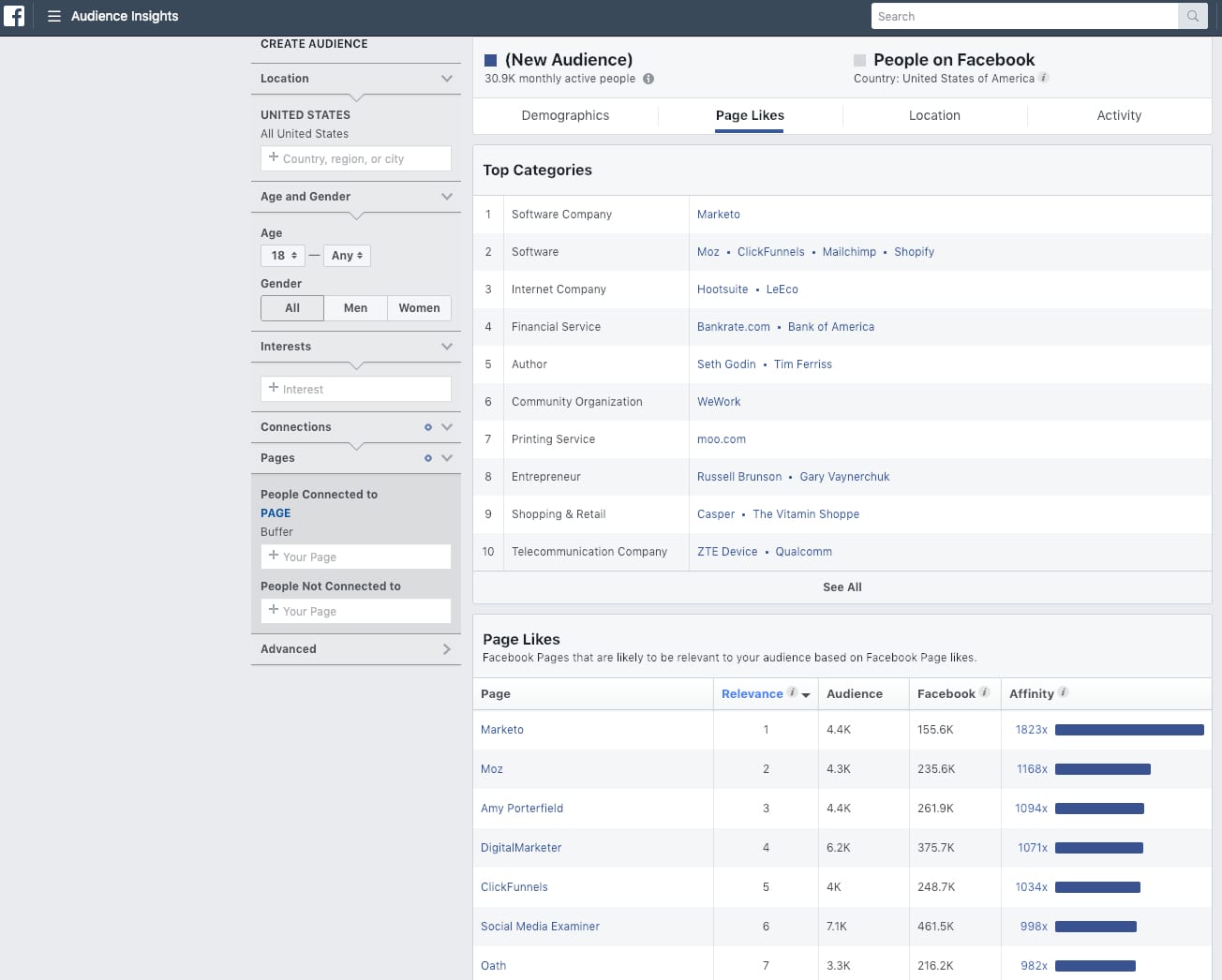The image depicts a webpage designed for audience insights, featuring a sophisticated black and white theme for enhanced readability. At the top of the page, a dark black box prominently displays the text "Audience Insights." Below this, a grey-toned box appears, housing the options for creating a new audience, with selections for location, age, gender, interests, and more. The dropdown menus and headers in this section are highlighted in blue for easy navigation.

On the upper right side, there's a search bar that is currently empty. Adjacent to this, the text "New Audience" is displayed. The webpage identifies "People on Facebook" in bold, dark black font, and further segments the audience by demographics, page likes, location, and activity.

One highlighted section, "Page Likes," discusses how certain Facebook pages are likely to be pertinent to your audience based on current page likes. It lists top categories that include terms such as "software company," "software," and "internet." Directly below, there is an option to view all categories. Each segment is crisply organized to provide comprehensive insights into audience analytics, making it easier for users to tailor their marketing efforts efficiently.